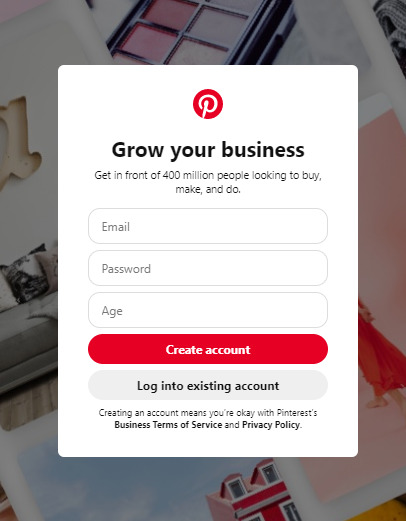The image depicts a Pinterest promotional page inviting users to grow their business by reaching over 400 million potential customers. The page's background features a serene arrangement including various make-up kits and face make-up sets, tastefully displayed on couches, with framed pictures adding a cozy ambiance. Central to the image is a prominent call-to-action encouraging users to get started. Below this message, there are empty fields prompting for email, password, and age input, flanked by buttons to create an account or log into an existing one. A subtle reminder at the bottom indicates that signing up implies agreement to Pinterest's business terms of service and privacy policy.